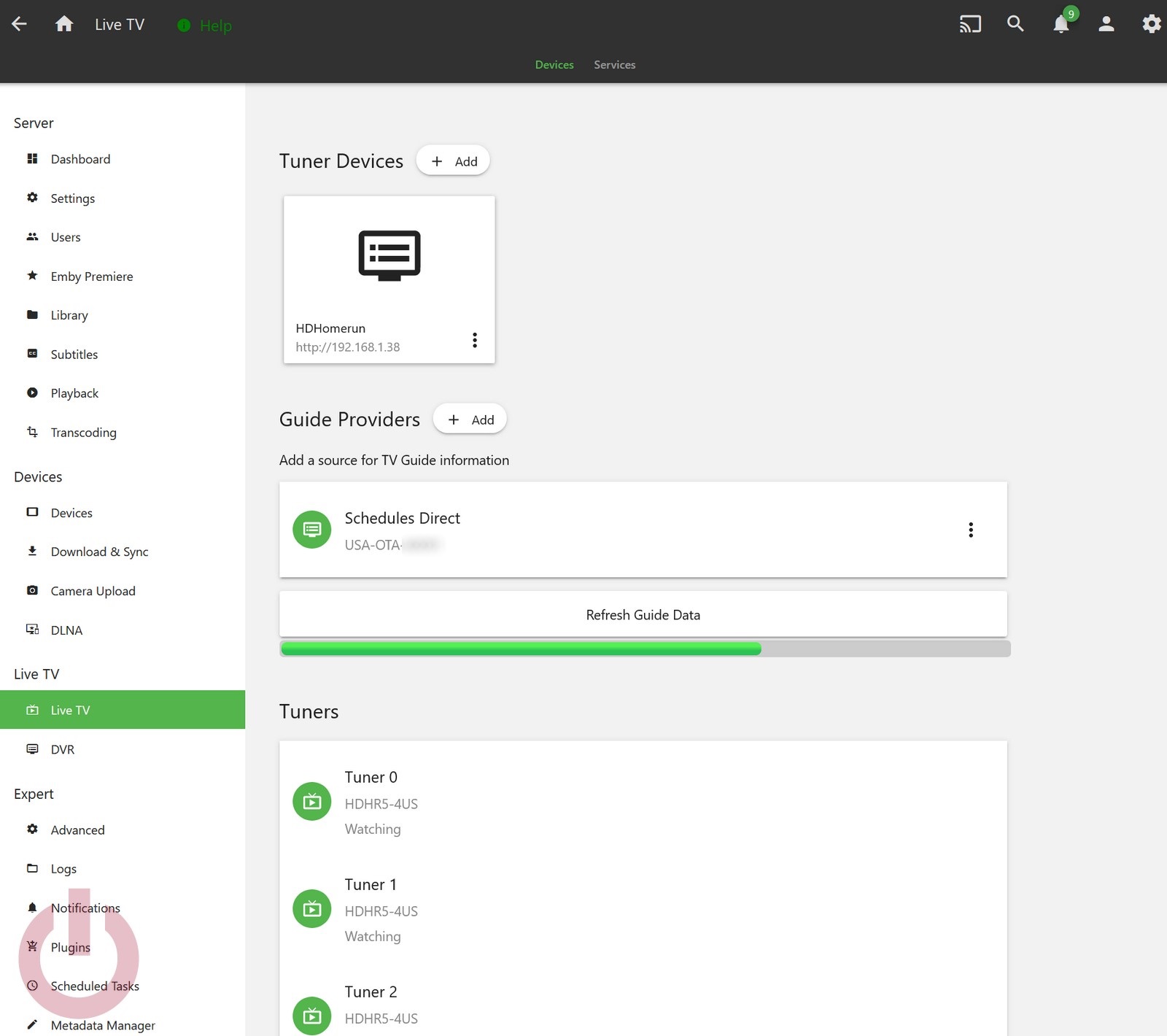Screenshot of a computer application interface showing a Live TV management window. The top of the screen features a black bar displaying navigation options and current directory information. On the left side of the interface, there is a vertical column with categories including Server, Dashboard, Settings, Users, Devices, Download Sync, and Live TV. The Live TV option is highlighted in green, indicating it is currently selected.

The main section of the screen displays several management boxes, including "Tuner Devices" and "Guide Providers." The "Tuner Devices" section shows multiple tuners labeled as Tuner 0, Tuner 1, and Tuner 2, with an icon for an HD Home Run device beneath it. The interface includes settings for different tuners and synchronization options.

At the top right, the black bar also contains icons for alerts, settings, profiles, and notifications, with a green bubble indicating nine unread alerts. The overall design features a darker gray background with sections of lighter gray and black font, providing a clear segregation of different functional areas within the application.